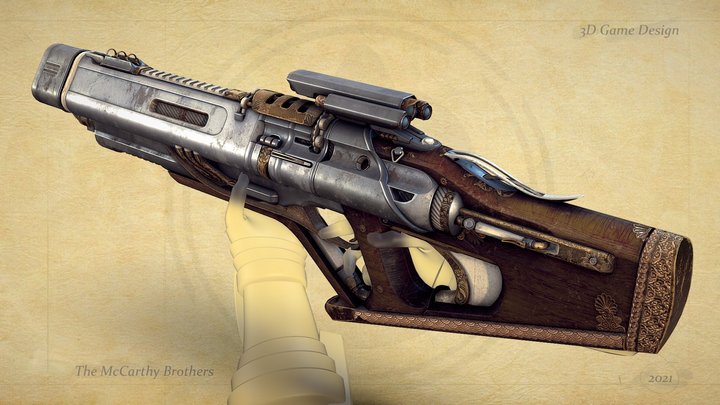In the image, we see an intricately designed, large steampunk-inspired gun with a mixture of metal and leather elements. The gun is predominantly silver with a wide, possibly spinning barrel that points towards the upper left corner of the image. The butt of the gun, made of wood or leather, rests against the right side of the weapon. A complex scope with three round sections is mounted on top. Supporting the gun is a translucent beige hand, holding it firmly from the bottom and another hand, partly visible, is gripping the trigger.

The background is a light brown, tan hue, resembling a vintage or aged paper texture. Below the gun is a structure resembling a pillar, providing a robust support base. The text "3D Game Design" is prominently displayed in the upper right corner, indicating the artistic and conceptual nature of the image. In the bottom left corner, the image is labeled with "The McCarthy Brothers" and in the bottom right, "2021," likely denoting the creators and the year of design. This highly detailed illustration suggests a concept for a video game weapon.